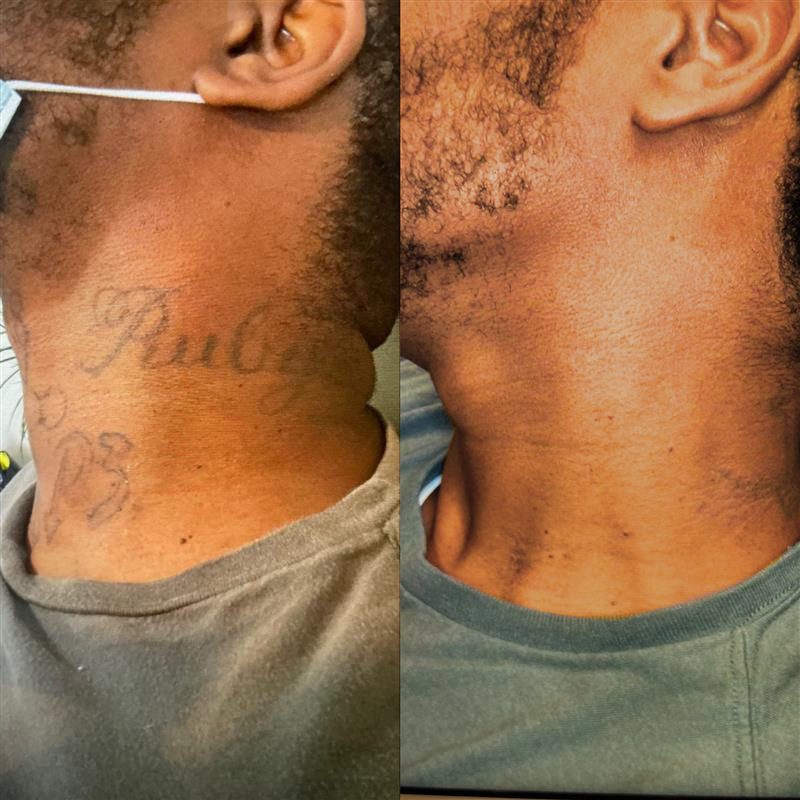In this image, we have two side-by-side, before-and-after photographs of a man's neck and lower face taken from a profile view, showcasing the left side of his face from around the ear down to the neckline of his green crew-neck shirt. The man appears to be of African-American or possibly another brown-skinned nationality. In the left photograph, which is the "before" shot, there are two semi-faded tattoos: one says "Ruby" in cursive letters on the neck, and another reads "P3" lower on the neck. Additionally, there is a faint line tattooed near his Adam's apple. In this image, he is also wearing a face mask, identifiable by the white elastic strap visible around his ear and the corner of the blue material. In the right photograph, the "after" shot, the tattoos have been removed, leaving his neck clear of any artwork. The face mask is no longer present but he is still wearing the same green shirt, indicating the photographs were taken in close succession.